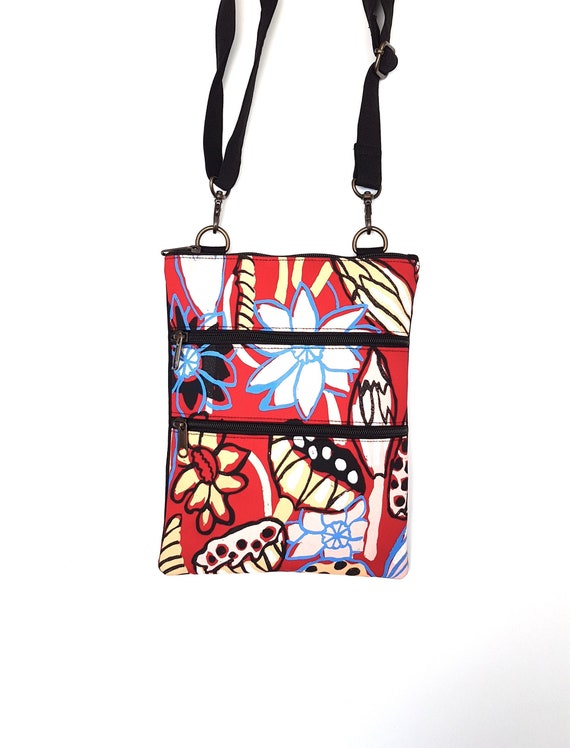The image depicts a vertically rectangular women's handbag adorned with a vivid red background featuring an intricate floral and mushroom design. The illustrations on the bag include various flowers, some outlined in blue and filled with white or black, while others are outlined in black and filled in with yellow. Notably, some flowers are depicted with black petals, and what appear to be mushrooms with teeth are also part of the artwork. The bag is taller than it is wide and is equipped with two silver rings at the top, to which a black strap is attached via spring-loaded clips. Additionally, it has two zippers running horizontally across the front, each leading to separate compartments. The zipper pulls are situated on the right-hand side of the image. The handbag rests on a white surface with some gray shading on the lower right, enhancing the depth and painting-like quality of the overall scene.